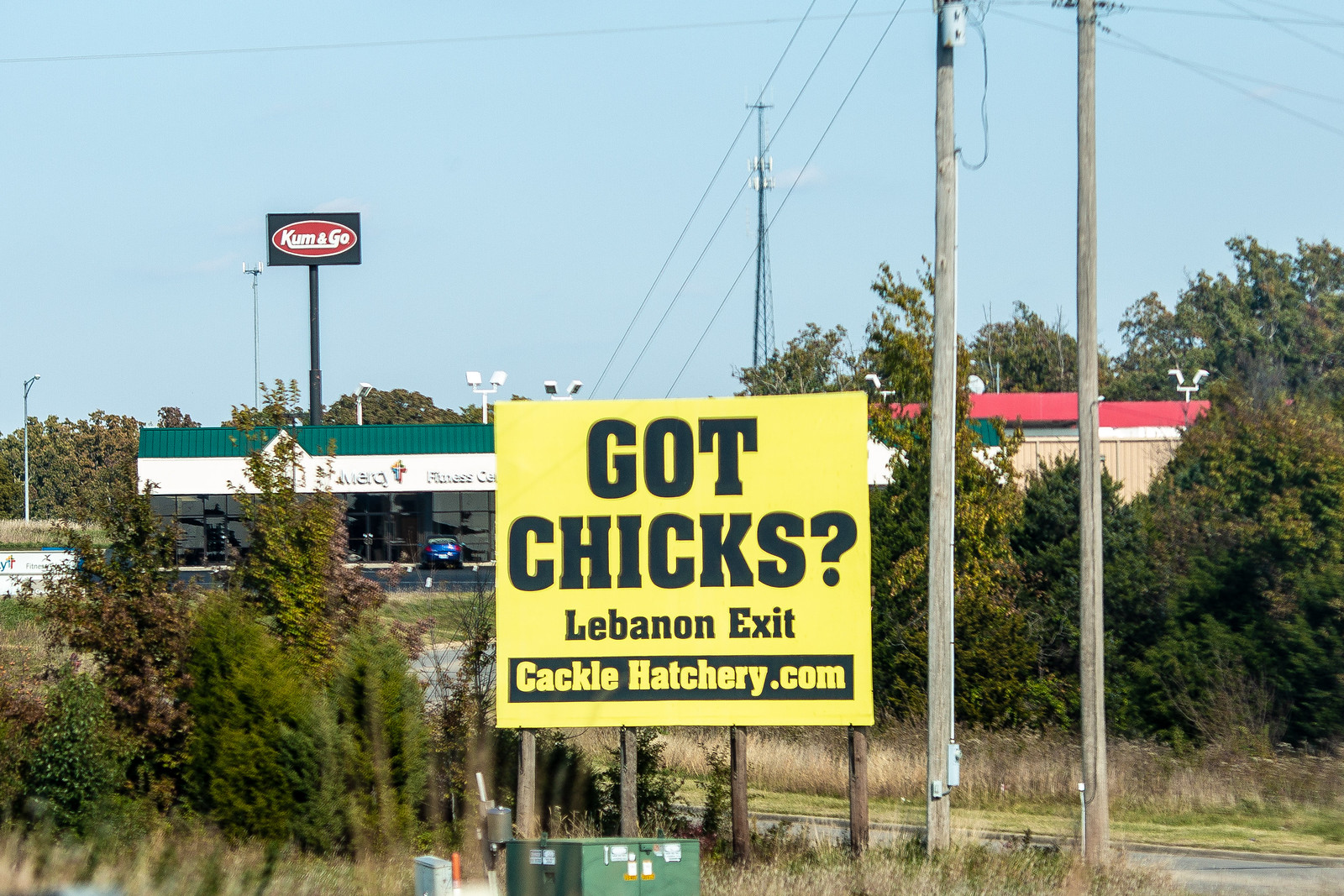The photograph captures a bustling urban scene centered around a large, prominent billboard with a yellow background and black text that reads, "Got Chix? Lebanon Exit, Cacklehatchery.com." This brightly-colored sign is mounted on four vertical posts and stands out against the surroundings. 

To the left of the billboard is a short vegetation area with scrubby, faded brown grass and a green square object that appears to be an electric box. Below this, there is a small office complex or strip mall with businesses that are hard to identify from this angle. A notable feature of this complex is a tall sign for a "Kum & Go" gas station, easily recognizable by the unique spelled name "K-U-M Ambersand Geo," which rises above the building. Below this sign, we see part of a parking lot with a blue car.

In the background, we can see another building with a red-colored roof, whose purpose is unclear—it may be a business or a residential property. To the right of the "Got Chix?" billboard are two wooden poles, presumably power or telephone poles, with three lines running vertically toward the left and right edges of the image. Additionally, a cell phone tower is visible far in the background, indicating an urban setting.

Overall, the image encapsulates a mix of urban development with businesses, advertisement, and essential infrastructure amidst a landscape of scrubby brown grass and sparse vegetation.